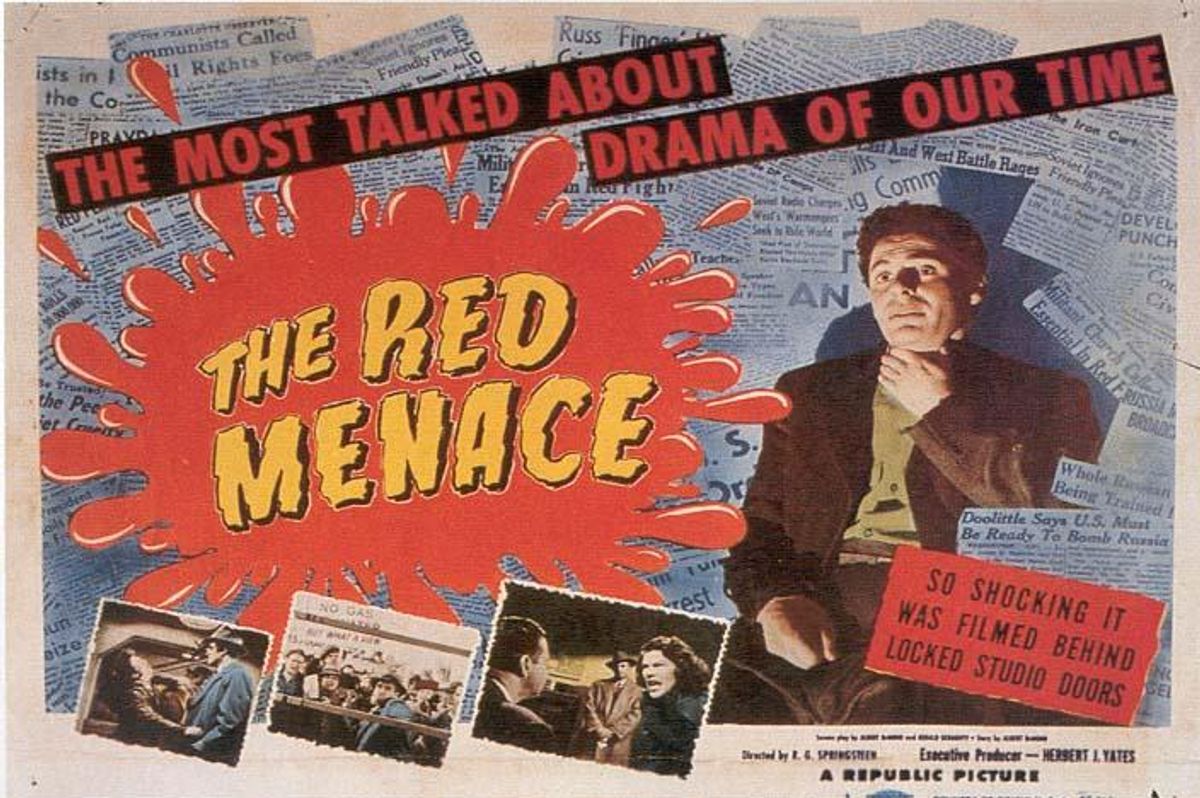This vintage movie poster, set within a horizontal rectangular frame with a light, almost beige background, features a compelling central design. At the heart of the poster, a smaller rectangular area is filled with an array of gray newspaper clippings, creating a collage-like texture adorned with black text. Diagonally crossing this textured background are two bold, black horizontal strips with striking red letters in capital font: the upper strip reads "THE MOST TALKED ABOUT" and the lower strip states "DRAMA OF OUR TIME."

Dominating the center-left of the poster is a large, dramatic red splatter that appears as if paint was vigorously thrown against the background. Contained within this vivid splash are the words "THE RED MENACE" in prominent yellow letters, making the film's title unmissable. To the right of this bold title, stands a concerned-looking white man with brown hair, dressed in a dark brown jacket over a light green shirt and matching brown pants, his left hand gripping his throat in a gesture of evident worry.

Beneath the central design, a red rectangular strip in the bottom right corner bears an alarming proclamation in black text: "SO SHOCKING, IT WAS FILMED BEHIND LOCKED DOORS." The lower section of the poster also includes cutouts of photographs, adding to the visual complexity and reinforcing the film's dramatic and mysterious allure.